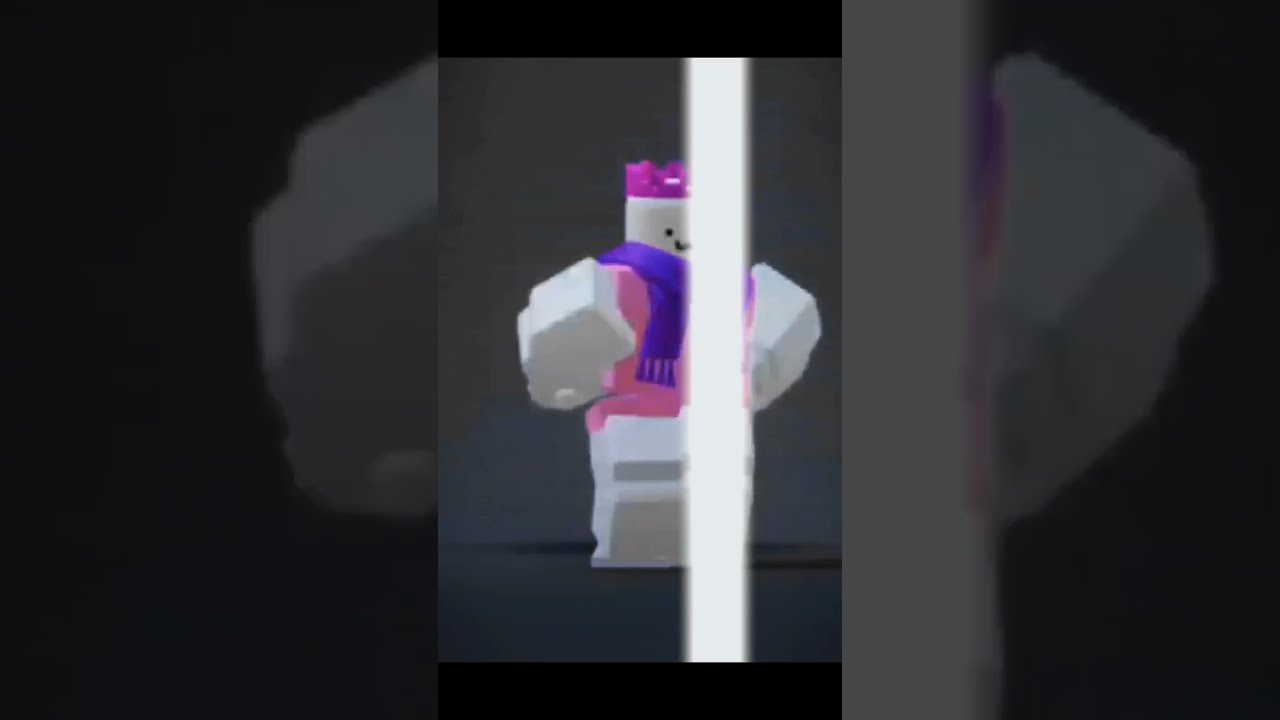The image depicts a scene divided into three vertical segments. The leftmost section is a dark gray blur with indistinct objects partially cut off by its right edge. The central segment, bordered in black on the top and bottom, features a cartoonish character resembling a Lego figure or a snowman. This character is predominantly white with large arms and legs, and wears a pink top, a blue scarf with purple tassels, and a purple crown on its head. The head displays a simple black smiley face. There is a white vertical beam that obscures part of the character's right shoulder, casting a shadow behind it, suggesting movement. The rightmost section is another blurry area with a gray beam and a partially visible gray object against a dark background. The composition and style suggest that the image might be a low-quality screenshot from a video game or a live streaming session showing character art.